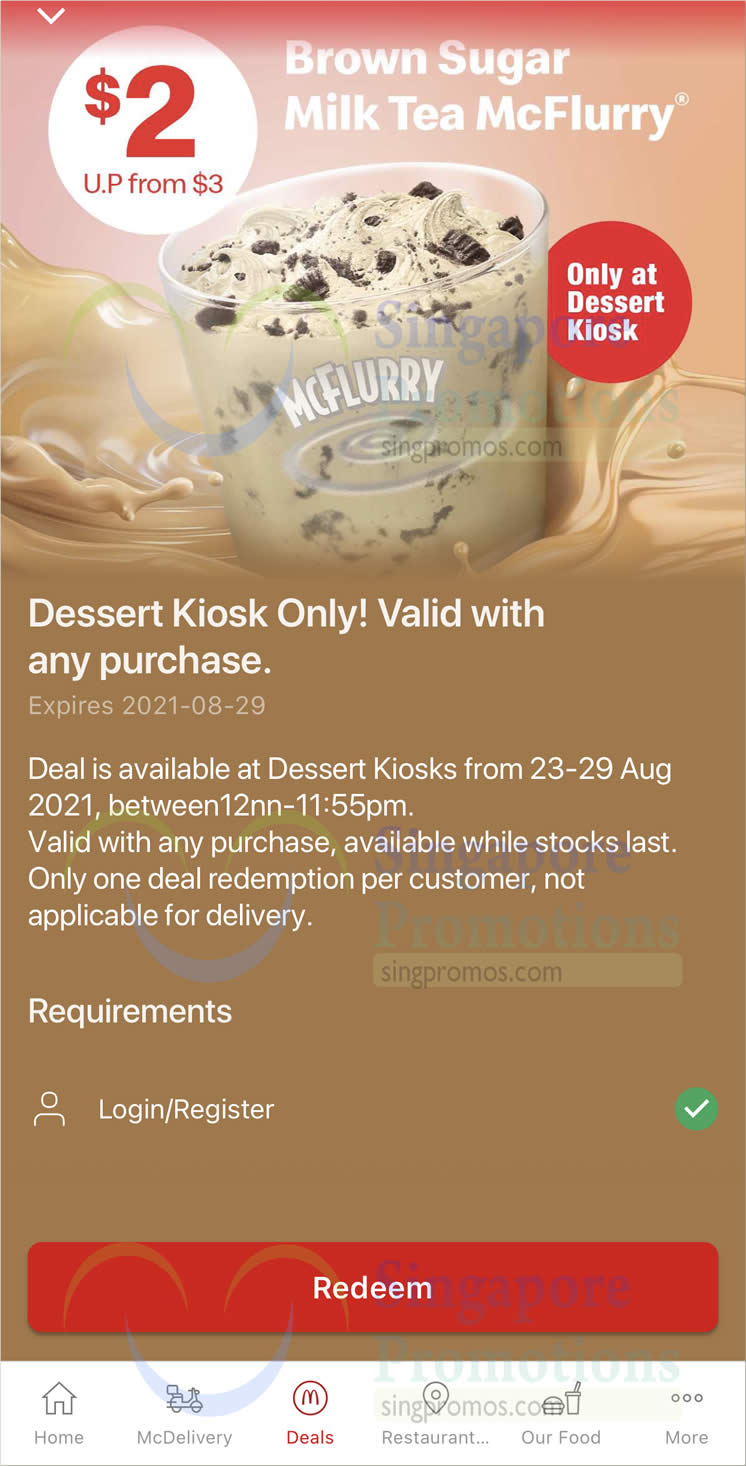**Descriptive Caption:**

In this promotional image, various elements and offers are neatly packed, revolving around the featured item: the Brown Sugar Milk Tea McFlurry. At the top right corner, against a slightly pink background, there is bold white text announcing the product's name, "Brown Sugar Milk Tea McFlurry." On the top left, the promotional price is highlighted; a white section with red text indicates, "$2 up from $3." 

The centerpiece of the image is a glass cup immersed in a rich brown chocolate backdrop. The cup contains a swirl of brown and black McFlurry ice cream and is emblazoned with the word "McFlurry" in white, outlined in grey.

Adjacent to the cup on the right side, a red area with white text specifies, "Only at Dessert Kiosk." On the left side, a detailed description in white text outlines the terms and conditions of the offer: "Dessert Kiosk only. Valid with any purchases. Expires 2021-2029. Deal is available at Dessert Kiosk from 23-29 August 2021 between 12 noon to 11.55pm. Valid with any purchase. Available while stock lasts. Only one deal. Redemption per customer. Not applied for delivery. Requirements. Login and register."

The bottom of the image features a red button labeled "Redeem" in white text, suggesting an actionable call to sign up for the offer. Below the button, several navigation tabs are present — "Home," "Melting Bar," "Deals" (highlighted in red), "Restaurant," and "Our Food Mall" in grey. 

The entire background is in red, with a watermark reading "Signed Promotion" subtly placed across the image. At the very bottom, the word "Singapore" is noted, indicating the promotional region.

Finally, a faint watermark of a website, “signpromos.com,” is present, reinforcing the promotional source.